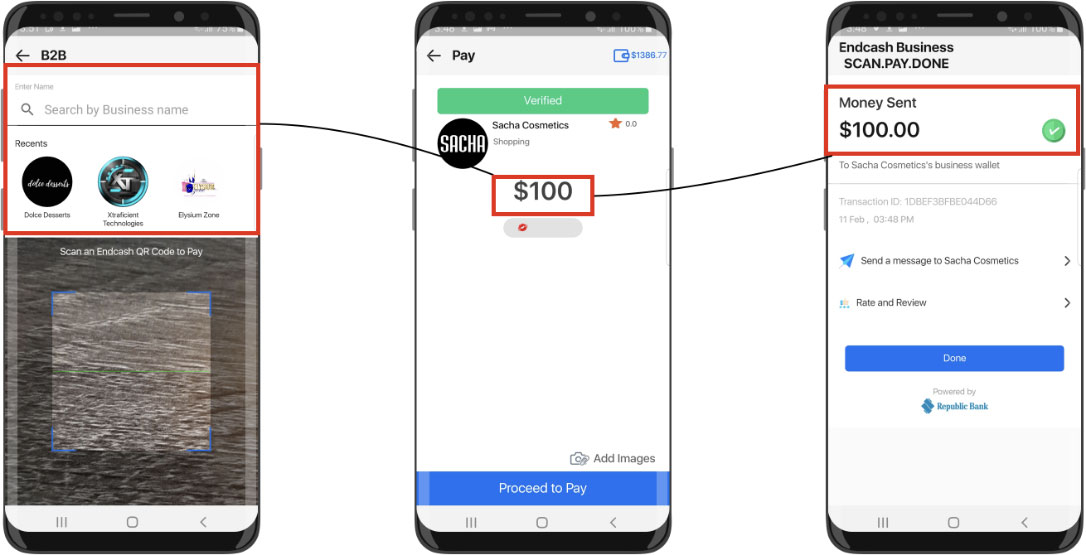The image features three cell phone screens, each showcasing different stages of a payment process for a business transaction. 

1. **First Screen (Left):** 
   - Displays a user interface with a red, horizontally elongated triangle at the top, containing the text "Enter Name" and a search icon.
   - Below, the text reads "Search by Business Name," followed by a section labeled "Recent" which lists businesses such as "Doluchi Desserts" and "Instant Technologies."
   - Despite the poor resolution, the screen is a search interface aimed at finding specific businesses.

2. **Second Screen (Middle):**
   - The focal point of this screen is a $100 amount enclosed in a red box.
   - The screen is titled "Sasha Cosmetics," indicating that the user has selected this business for a monetary transaction.
   - This screen represents the review of the payment amount before proceeding.

3. **Third Screen (Right):**
   - It confirms the transaction, displaying an interface with the text "Money Sent $100."
   - A green circle with a white checkmark signifies a successful payment.
   - Additional text "To: Sasha Cosmetics Business Wallet" details the recipient of the funds.

Thin black lines connect the red-outlined sections between each screen, illustrating the logical flow from searching for a business, reviewing the payment amount, and confirming the transaction. This sequence serves as a learning tool, guiding users through the steps of initiating and completing a payment to a business using a mobile application.